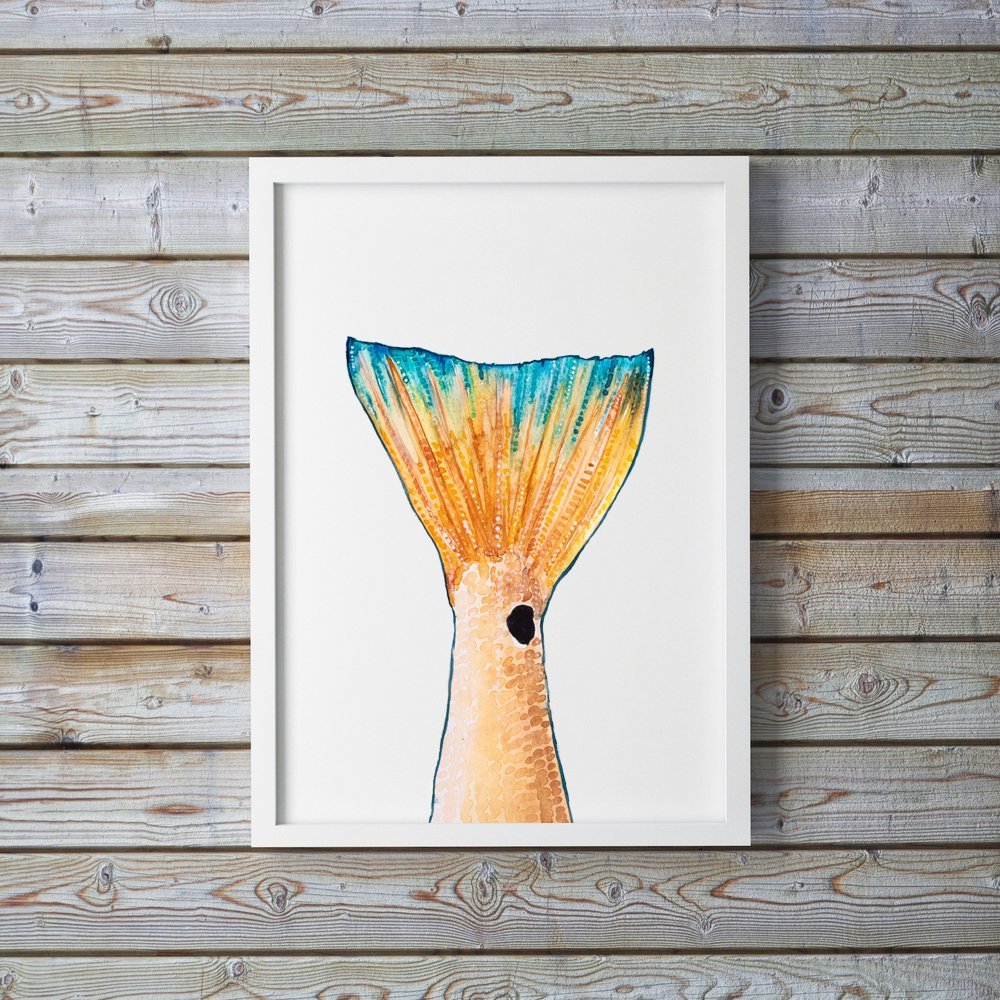The image features a framed piece of art displayed on a wall made of horizontal wooden planks with visible wood grains, knots, and a grayish, light brown tan color. The picture frame is white, with a white background. At the center of the frame, the art depicts only the tail of a fish. The tail has a vibrant turquoise blue tip, transitioning to peach and orange tones in the main body. Additionally, there is a single black dot near the base of the tail, adding a focal detail to the composition. The fish scales closer to the base are lighter peach, with some areas showing a light brown tan color.